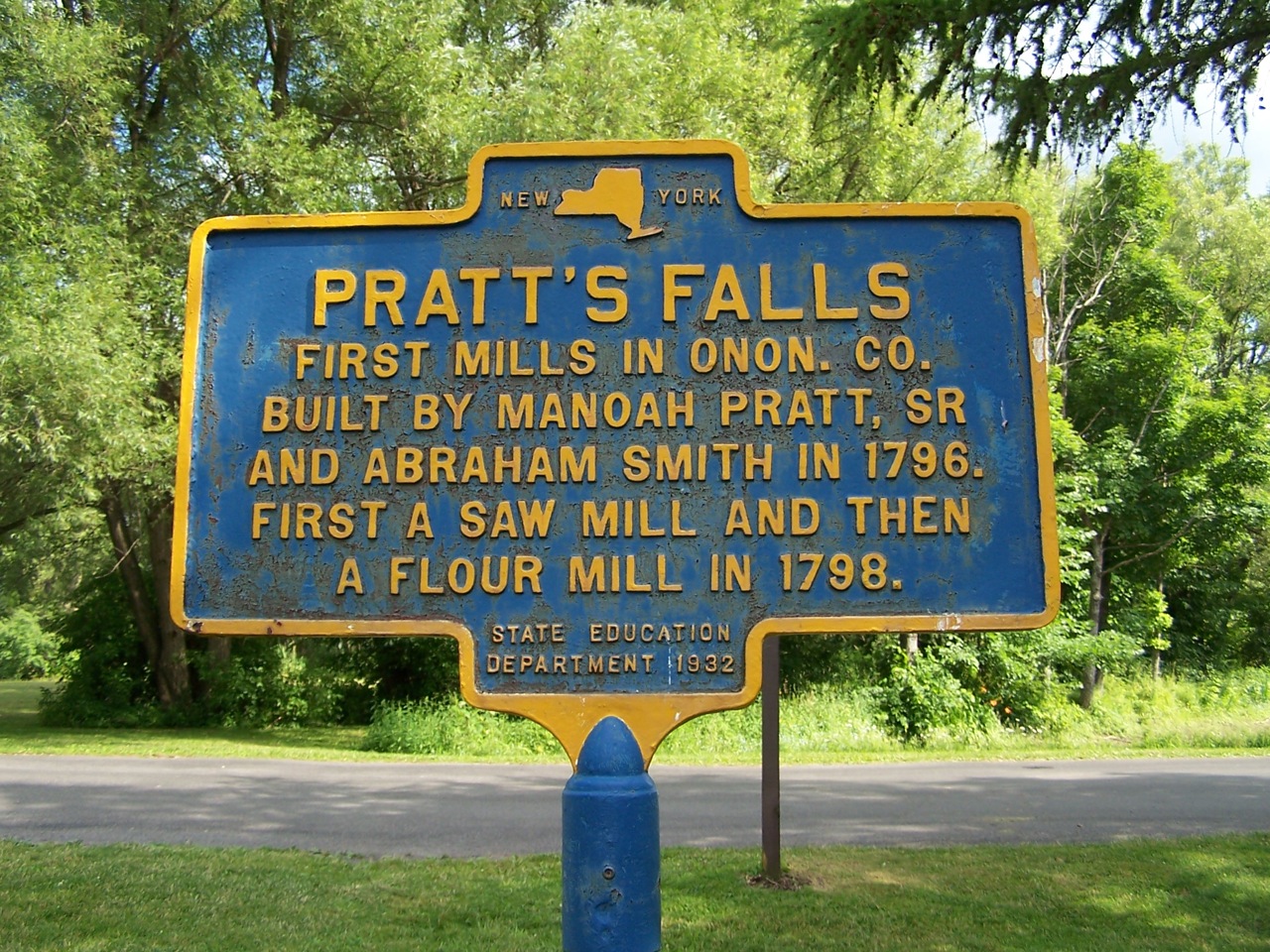The image depicts an old, weathered metal sign, mounted on a blue post with noticeable rust spots, situated in front of a backdrop of tall, leafy green trees. The sign has a unique shape, resembling a rectangle with square bumps at the top and bottom. It features a yellow border and text, with predominant blue and orange hues. At the top, it reads "New York" with a silhouette of the state between the words. The main text highlights "Pratt's Falls," noting that the first mills in Onondaga County were built by Manoa Pratt Sr. and Abraham Smith in 1796, starting as a sawmill and later adding a flour mill in 1798. The sign, a product of the State Education Department in 1932, shows significant signs of aging, with peeling paint and rust. Below the sign, there is a light gray pathway with tree shadows cast across it, adding to the historic and natural ambiance of the scene. To the right of the sign, another rusted post is partially visible, enhancing the rustic aesthetic of this historical marker.